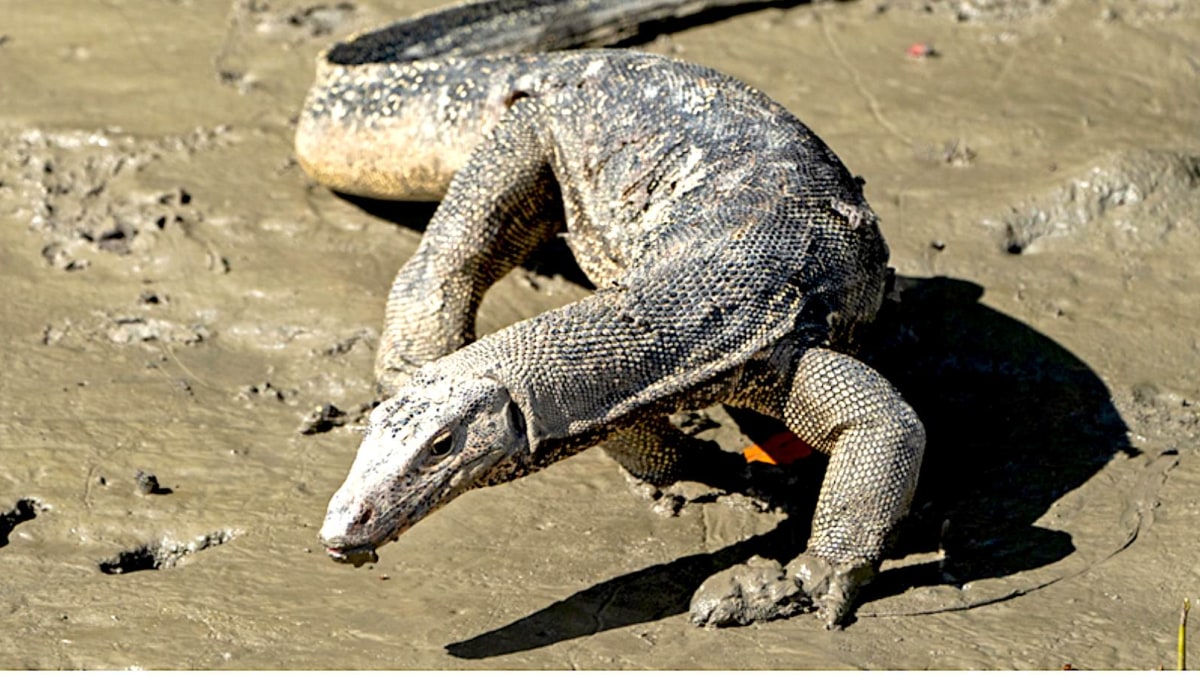This close-up photograph captures a giant lizard—most likely a monitor lizard—moving through wet, shiny mud. The lizard, resembling both an alligator and a dragon with its scaly, narrow head, and thick, elongated body, dominates the center of the image. Its head points towards the lower part of the photo while its body extends upwards, partially out of view. The scales, varying from dark gray to light gray, appear to be shedding in parts, indicating molting. The head has a lighter gray to almost white color, contrasting its black eyes and closed mouth. The lizard's thick, powerful arms and short legs are partially submerged in the light to dark brown mud, which visibly coats its feet. The underbelly of the lizard shows a lighter hue, ranging from light green to white. The scene is rich in texture, with the lizard seemingly wobbling as it walks through the slick, muddy terrain, possibly on the hunt for food.